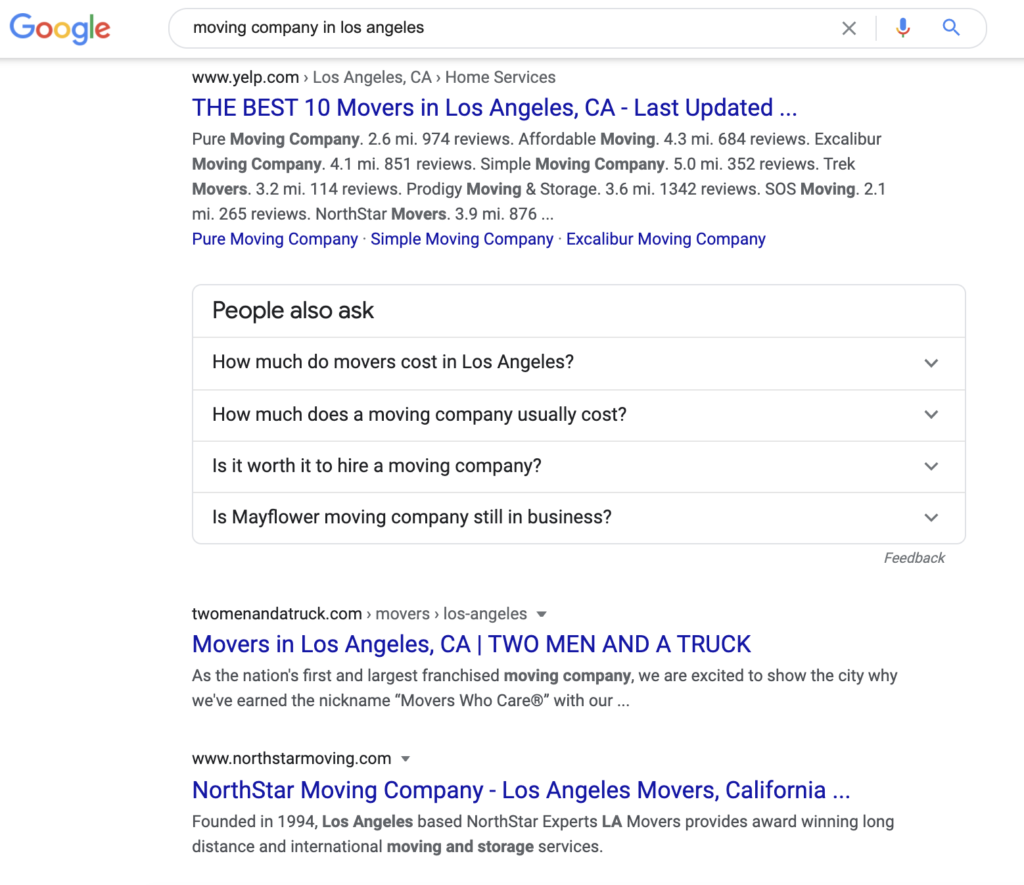A screenshot of a Google search displays results for "moving company in Los Angeles" with the headline "10 best movers in Los Angeles, California." The search also includes the "People also ask" section, featuring common questions such as "How much do movers cost in Los Angeles?" and "Is it worth it to hire a moving company?" Notable moving companies listed include Pure Moving Company, Simple Moving Company, Excalibur Moving Company, Two Men and a Truck, NorthStar Moving Company, and Mayflower Moving Company. The clickable links are highlighted in blue, while standard text appears in black. This visual layout clearly distinguishes between various options and related inquiries, offering a user-friendly interface for those searching for reliable moving services in Los Angeles.